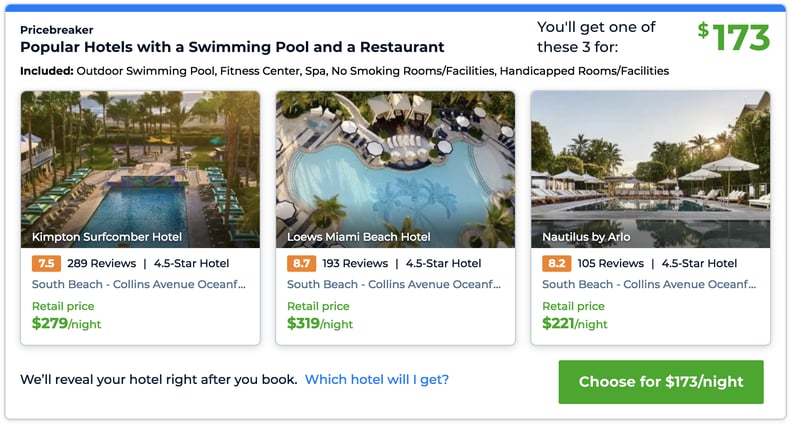**Detailed Caption:**

The image appears to be a screenshot from a hotel booking website or app. The interface has a tan and blue banner at the top, with black text on a white background that prominently reads "Price Baker." Below, the text indicates that you can book one of three popular hotels, each offering amenities like a swimming pool and restaurant, for a price starting at $173. The details mention included amenities such as an outdoor swimming pool, fitness center, spa, non-smoking rooms, and facilities for handicapped guests.

The page showcases three hotel options with corresponding images and details:
1. **Kingston Somerford Hotel**: Located on the left side, the image features a swimming pool surrounded by trees. The hotel has a 7.5 rating based on 289 reviews and holds a 4.5-star rating. The location is South Beach, Collins Avenue, with a retail price of $279 per night.
   
2. **Lowe's Miami Beach Hotel**: In the middle, the image also displays a swimming pool scene. This hotel boasts an 8.7 rating from 395 reviews and a 4.5-star rating. Situated in South Beach, Collins Avenue, it has a retail price of $379 per night.
   
3. **Nautilus by Arlo**: On the right, the picture shows a pool flanked by trees and umbrellas, with a glimpse of blue sky. It has an 8.2 rating based on 105 reviews and is rated at 4.5 stars. This hotel is also located on South Beach, Collins Avenue, and the retail price is $221 per night.

The site indicates that your specific hotel will be revealed after booking, making the process somewhat like a lottery. You can choose to book any of these three hotels at the rate of $173 per night.